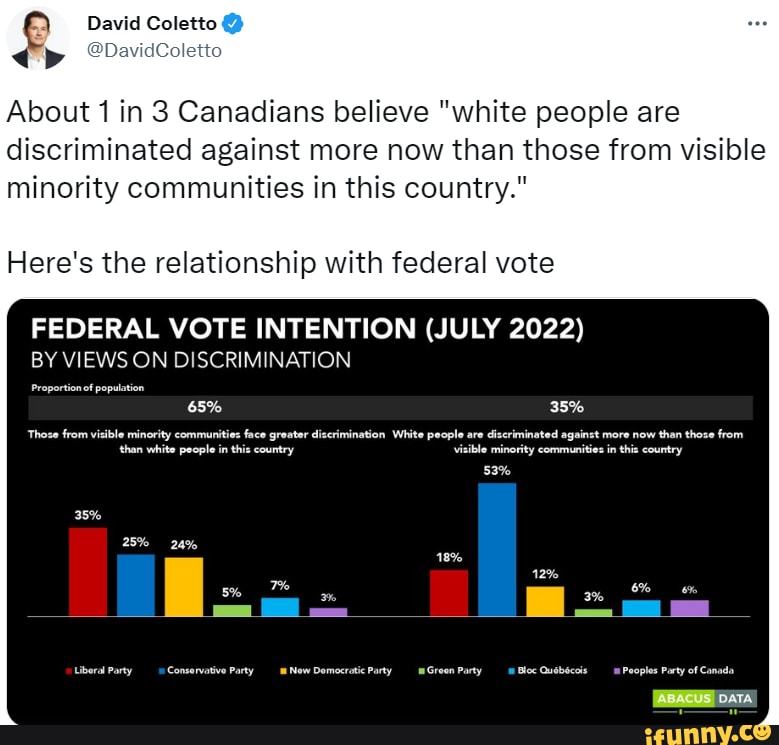The image is a detailed close-up of a tweet by David Coleto, who is verified and has a profile picture of himself looking into the camera while wearing a black-grey suit coat over a white shirt, sans tie. David has short black hair. 

The tweet reads: 

"About 1 in 3 Canadians believe white people are discriminated against more now than those from visible minority communities in this country."

Beneath the tweet, there's a space followed by a line that says:

"Here's the relationship with federal vote."

Below this line is a black box featuring bar graphs that are labeled "Federal Vote Intention, July 2022" with a specific focus on "By views on discrimination." The bar graphs inside provide numerical data illustrating federal voting intentions segmented by perspectives on discrimination.